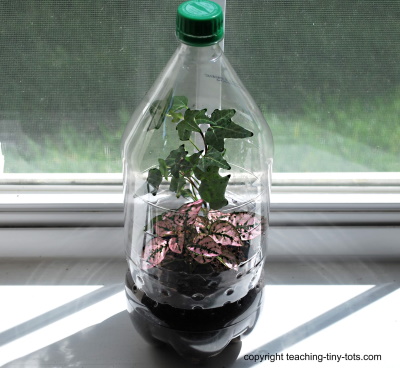In this close-up color photograph, a repurposed two-liter clear plastic soda bottle, with its label removed and a green screw cap, has been transformed into a mini terrarium. It sits on a windowsill, basking in the sunlight streaming through the window, which highlights the lush green lawn visible outside through the screen. The bottle is cut around the middle and taped back together, allowing for air circulation with holes poked into it. Inside, the bottom of the terrarium is filled with dark soil, nurturing two types of plants: a vibrant green ivy and a Bidium plant with striking pink and green leaves. At the bottom right corner of the image, the text "copyright teaching-tiny-tots.com" is written in all lowercase.